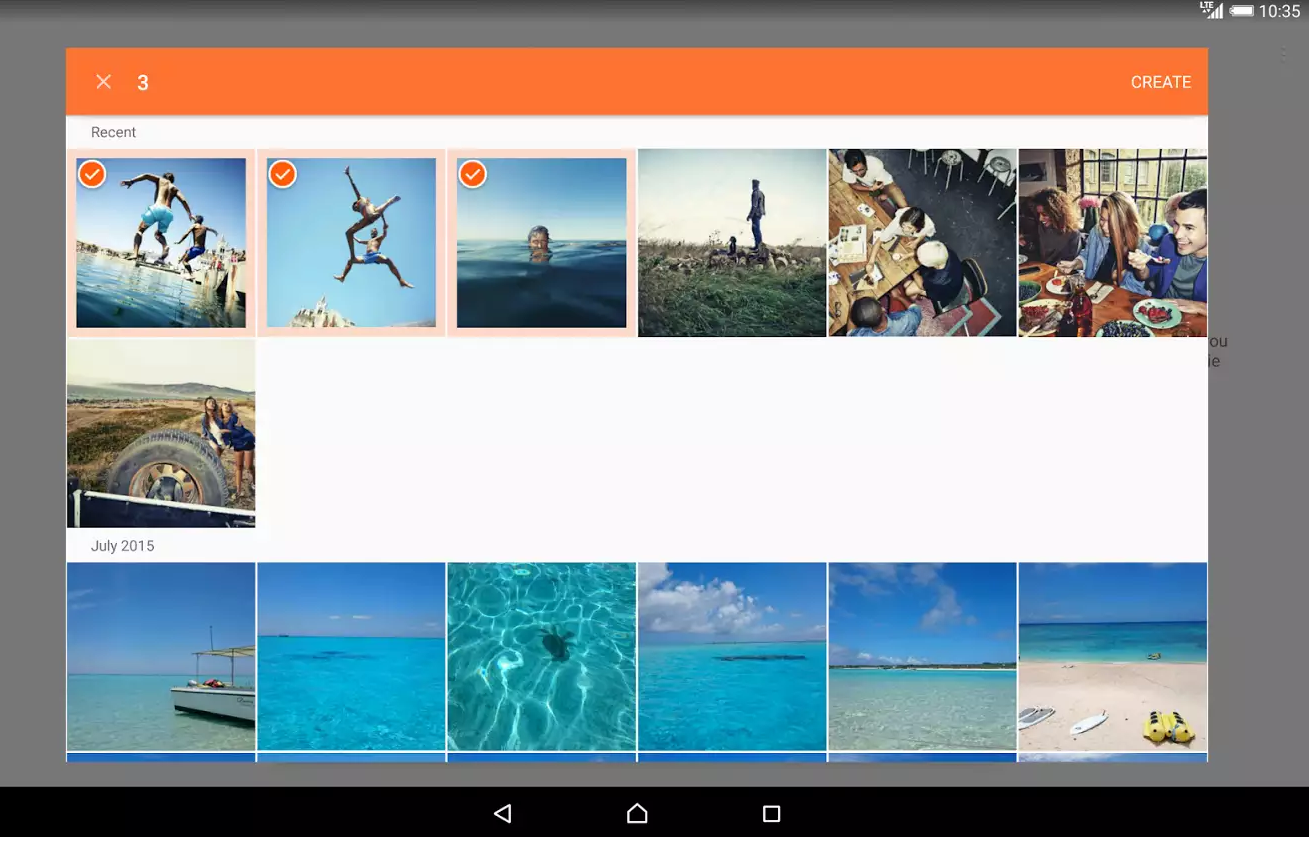A collage of multiple outdoor images enjoying the ocean is displayed. The collage is organized into three rows. The first and last rows each contain six images, while the middle row has only one image. The first row is labeled 'Recent,' and the first three images in this row are highlighted with a pink box around them. Within each of these three highlighted images, there is an orange circle with a white check mark in the top left corner. 

In detail:
- The first image shows two guys mid-air, seemingly jumping into the water.
- The second image features two individuals, possibly also jumping, with one person distinctly wearing blue shorts.
- The third image captures a single person in the water.

The remaining images on the first row, as well as those in the middle and last rows, continue the theme of outdoor enjoyment, potentially featuring various activities related to the ocean.